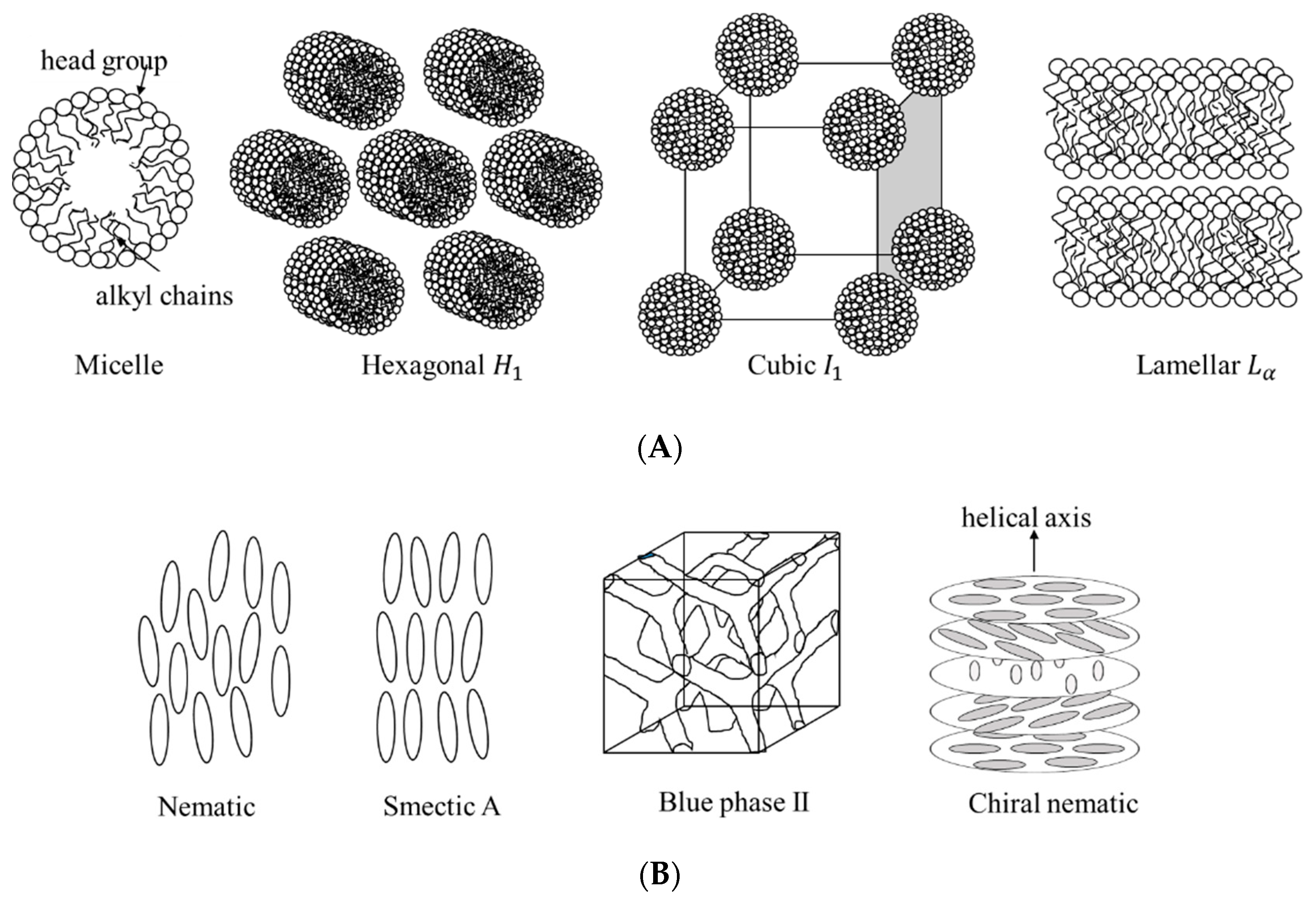The image is a black-and-white diagram illustrating eight different structures, evenly split into two rows. The upper row, labeled as 'A,' features four different molecular configurations: From left to right, the first diagram shows a 'Micelle,' depicted as a circular arrangement of small balls labeled as the 'head group' with lines representing 'alkyl chains' radiating outwards. The second diagram is titled 'Hexagonal H₁,' showing stacked hexagonal tubes. The third is 'Cubic I₁,' illustrating a cubic structure, followed by 'Lamellar Lα,' depicting layered, parallel sheets. 

The bottom row, labeled as 'B,' also has four diagrams: the first is 'Nematic,' with loosely arranged ovals, followed by 'Smectic A,' displaying aligned ovals. The third in this row is 'Blue Phase II,' characterized by a complex, cubic arrangement resembling antlers. The final diagram is 'Chiral Nematic,' again showing organized structures but with a twisted, helical pattern. Each diagram shows different molecular organizations and phases, providing a detailed comparison of these distinct formations.